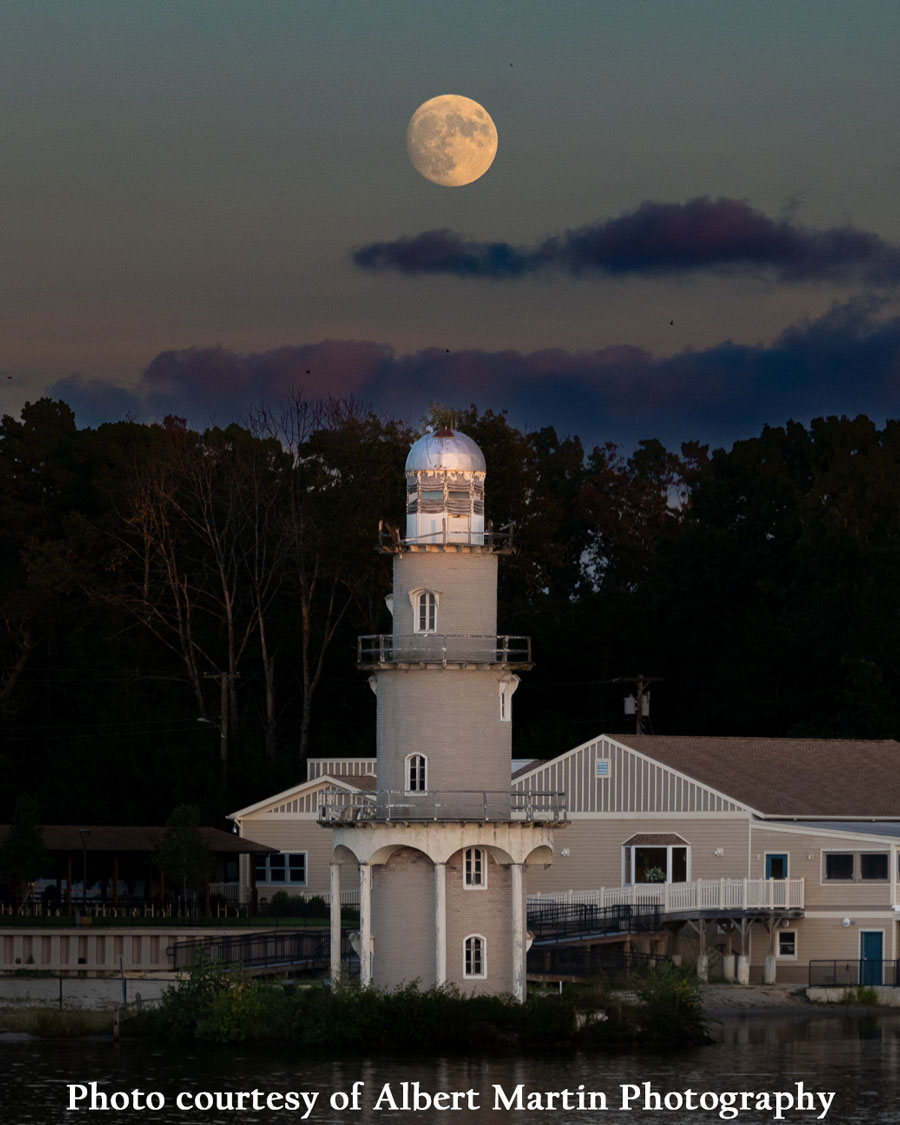This detailed photograph, titled "Photo Courtesy of Albert Martin Photography," features a modern lighthouse seamlessly connected to a beige building, possibly serving as a lodge, bed and breakfast, or residence. The lighthouse, with its light beige exterior and white trim, stands tall with four distinct stories. The first level is supported by stone columns, followed by multiple windows on each tier, some featuring balconies. The top of the lighthouse is capped with a clear dome where the light emanates, though it appears dim in the image. The accompanying building, matching the lighthouse in color, includes green doors, several balconies, and a sheltered area with a car. A walkway with a railing extends from the lighthouse, connecting it to the rest of the structure.

In the background, large trees create a dark silhouette against the sky. The night sky is partly cloudy with streaks of purple and pink clouds framing a nearly full moon positioned directly above the lighthouse. To the left, a white fence and ramp add to the picturesque setting. The photo captures a serene and mystical evening scene, highlighting the harmonious blend of architecture and nature.